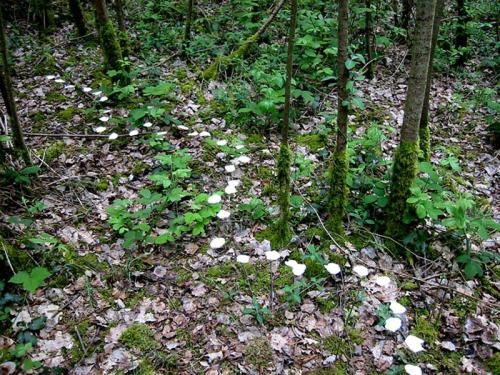This is an aerial photo taken in a forested area, featuring a cluster of slender, moss-covered trees primarily centered and slightly off to the right. The forest floor is a mix of green and decaying ground cover, creating a lush, yet varied landscape. There is a distinctive linear path formed by evenly spaced white splotches or circles—possibly mushrooms or flowers—that meander from the bottom right corner, snaking through the frame and eventually extending diagonally to the top left. The light filtering through the canopy is soft and even, enhancing the visibility of the intricate details on both the mossy trunks and the various foliage scattered across the ground. The overall composition suggests a serene and slightly mysterious natural setting.